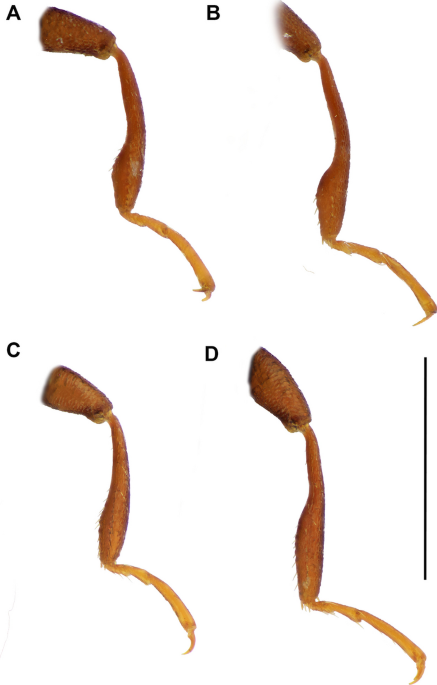The image showcases four similar-looking insect limbs, possibly belonging to an ant or scorpion, labeled A, B, C, and D. All limbs share a goldish-brown, slightly see-through coloration and are depicted against a white background. These limbs are mostly the same size but exhibit minor variations, with D being noticeably larger than C. The limbs are detailed with small hairs and end in distinctive claws: A has two small claws, B has a single claw, C has a raptor-like claw, and D features a larger raptor-like claw. This detailed depiction, suitable for a scientific publication, highlights both the similarities and differences in the limb structures.